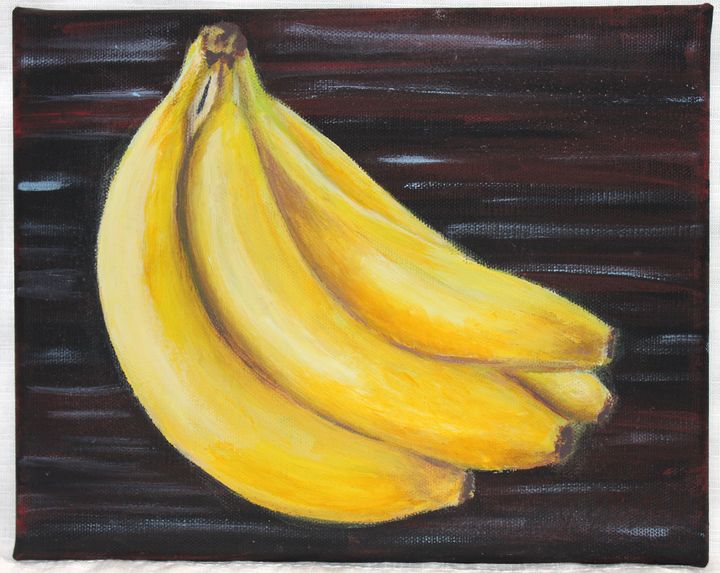This rectangular image, which has the appearance of a painting, prominently features a ripe, golden-yellow bunch of four bananas. The bananas are clustered together by their stems, displaying a slight touch of green at the top stem and dark brown hues at the tips. The background contrasts starkly with the vibrant yellow of the bananas, presenting an artistic pattern of alternating stripes in black, maroon, and blue shades, reminiscent of a wood-like texture. This visually stimulating backdrop is bordered by a subtle gray frame that further enhances the overall depth and dimension of the artwork. The detailed shading and color variation in the bananas highlight their freshness and ripeness, creating a striking focal point against the textured, multicolored background.